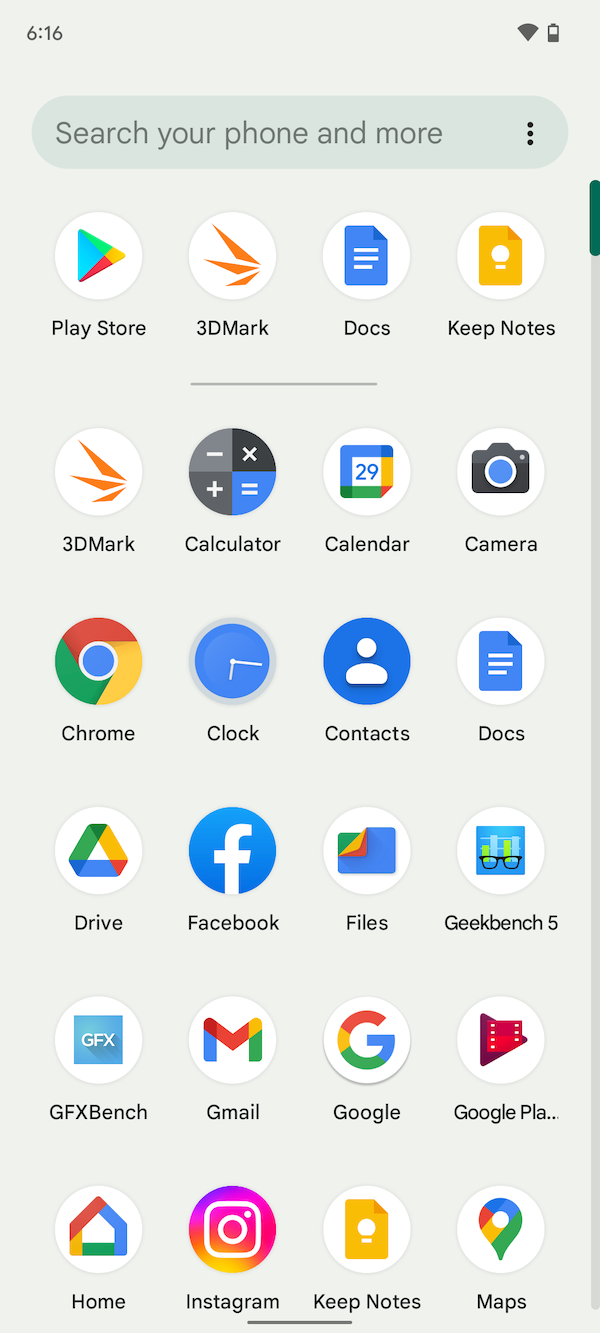This image captures a screenshot of a mobile phone's application page, characterized by a grey background with a slight greenish hue. In the top left corner, the screen displays medium grey text reading "616," while the top right corner houses two icons: a fully dark grey Wi-Fi icon and a half-full dark grey battery icon.

Beneath these icons, a slightly darker grey search bar, tinged with green, spans the width of the screen. It contains large, medium grey text stating "search your phone and more," and is accompanied by three vertically stacked black dots on its right.

Below the search bar, the screen features rows of circular app icons. The top row consists of four icons with white backgrounds, each labeled in dark grey text beneath: Play Store, 3D Mark, Docs, and Keep Notes. A thin medium grey line, centered and matching the width of the two central icons, separates the top row from subsequent rows.

The following rows display four app icons per row, with labels as follows (from left to right and top to bottom): 3D Mark, Calculator, Calendar, Camera, Chrome, Clock, Contacts, Docs, Drive, Facebook, Files, Geekbench 5, GFXBench, Gmail, Google, Google Play, Home, Instagram, Keep Notes, and Maps.

A scrollbar on the right edge of the page runs nearly the entire height of the screen, featuring a small, green, vertical pill shape at the top indicating the current scroll position.